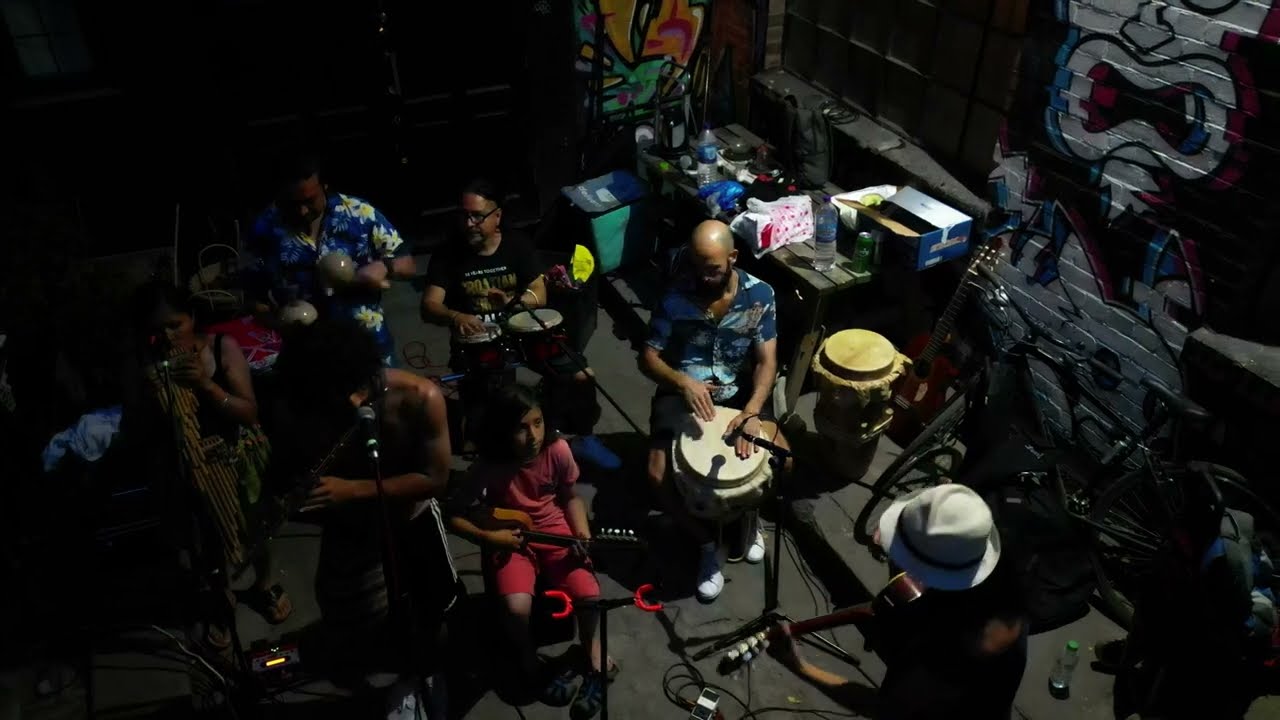This image is an aerial view of a dimly lit room, likely a bar or concert venue, where several musicians are gathered, playing various instruments. The central and left portions of the image show the musicians more clearly, while the top left is shrouded in darkness.

On the top left, a man in a blue and yellow Hawaiian patterned shirt energetically shakes two brown maracas. Next to him, slightly to the right, a man with black glasses, dark hair, and a black t-shirt with a pattern, is seated and playing red bongos that rest on his lap. To his right, a bald man wearing a blue Hawaiian shirt is focused on a drum positioned between his legs.

In front of these three, a younger person with dark black hair, dressed entirely in red, strums a small ukulele or guitar, adding a string melody to the ensemble. To the left of this young musician, another person plays an unidentified instrument, but they are obscured by shadows and dressed in dark clothing, making them difficult to distinguish. Further left, a woman with dark hair is seated, playing brown panpipes that contribute a soft, airy sound to the music.

The right side of the room's wall features a vibrant, graffiti-styled mural in blue, red, and white, with cartoon-like characters. Near the center-right of the image, a cluttered dark wooden table is visible, covered with various objects, boxes, and clear plastic water bottles. The floor is a dark gray, adding to the room's dimly lit atmosphere.

Amidst the subdued lighting, a second light source from the back top right appears to highlight some areas more prominently, creating pockets of visibility within the dark ambiance of the room.